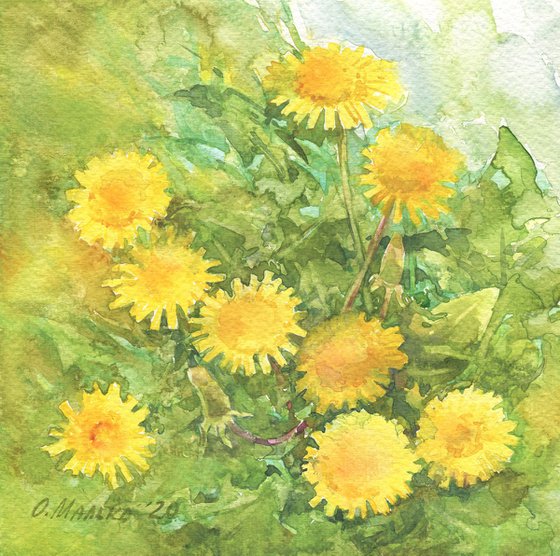This painting, done in watercolors on watercolor paper, features a vibrant collection of yellow flowers that resemble sunflowers, although some descriptions suggest they might be dandelions. The painting is perfectly square, with dimensions that emphasize its symmetry. The background is a blend of loose shades of greens, blues, and whites, blending seamlessly with the flowers, creating a soft, splotchy texture typical of watercolor art. 

At the forefront are nine sunflowers, each about the size of a dime, characterized by their rectangular petals arranged in a circular formation around fuzzy yellow centers. Some flowers are fully open, while others are budding. They are surrounded by a variety of stems and tall, pointed green leaves that range in color from dark green to lime green, with some stems showing hues of reddish-purple. The upper right corner of the background transitions into a lighter area with white smudges and hints of light green, evoking a sense of light and airiness.

The delicate detailing extends to the artist's signature in the lower left corner, faintly inscribed in black or possibly darker orange. The signature appears to read "O. MarLko, '20" or "O. Maalks, '20," though the exact lettering is somewhat unclear. Overall, the painting exudes a tranquil, natural beauty through its soft, watercolor technique and the harmonious depiction of flowers and foliage.